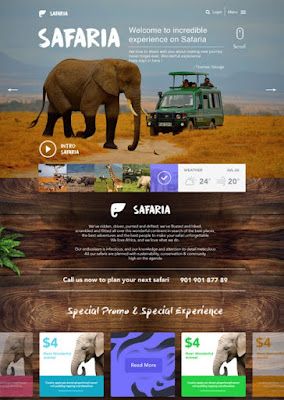The advertisement for an exciting safari adventure prominently features an outdoor scene under a clear blue sky. A majestic mountain, slightly blurred, forms the serene backdrop. In the foreground, an outdoor recreational vehicle, resembling a hybrid of a truck and an SUV, showcases a distinctive raised roof and a protective canopy. Walking gracefully in front of the vehicle is a stunning elephant, symbolizing the wildlife you can expect to encounter.

Across the middle of the advertisement, a vibrant banner displays illustrations of various animals you may spot on the safari, including a giraffe and a rhinoceros. Below the banner, a wooden panel background provides a rustic frame for a detailed line drawing of an elephant's head, notable for its trunk but missing the ears.

The bold text on the advertisement reads "Safari," followed by a call to action, "Call us now to plan your next safari," along with the contact number, 901-901-877-89. The ad invites you to take advantage of special promotions and promises a unique and unforgettable safari experience.